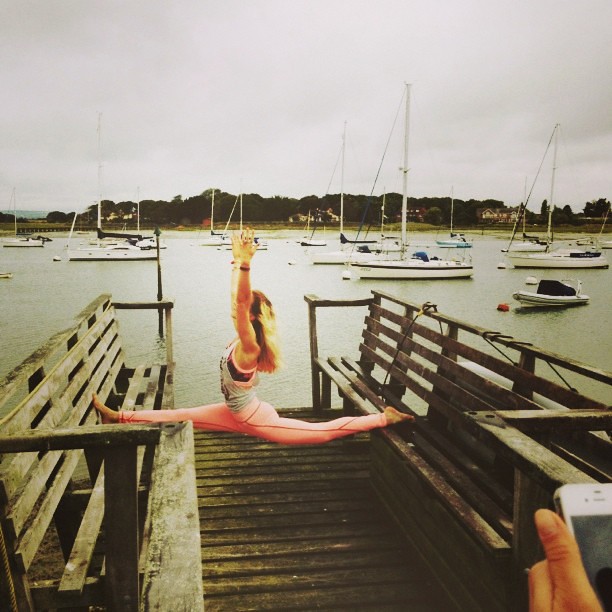In this striking color photograph, a young, fit woman with long blonde hair is captured mid-split, performing an impressive pose at a marina. She is dressed in a pink and white tank top paired with pink yoga pants, emphasizing her athletic form. The split is executed mid-air, with her right leg stretched forward on one weathered, eight-foot-long wooden bench and her left leg extended behind her on another bench, both positioned along a weather-beaten wooden pier. The background shows a gray sky over a large body of water, possibly a lake, dotted with anchored sailboats. Dark trees and four large waterfront homes add depth to the scene. A hand holding a smartphone in the bottom right corner suggests someone is photographing this moment, likely captivated by the serene yet powerful display of flexibility and strength.